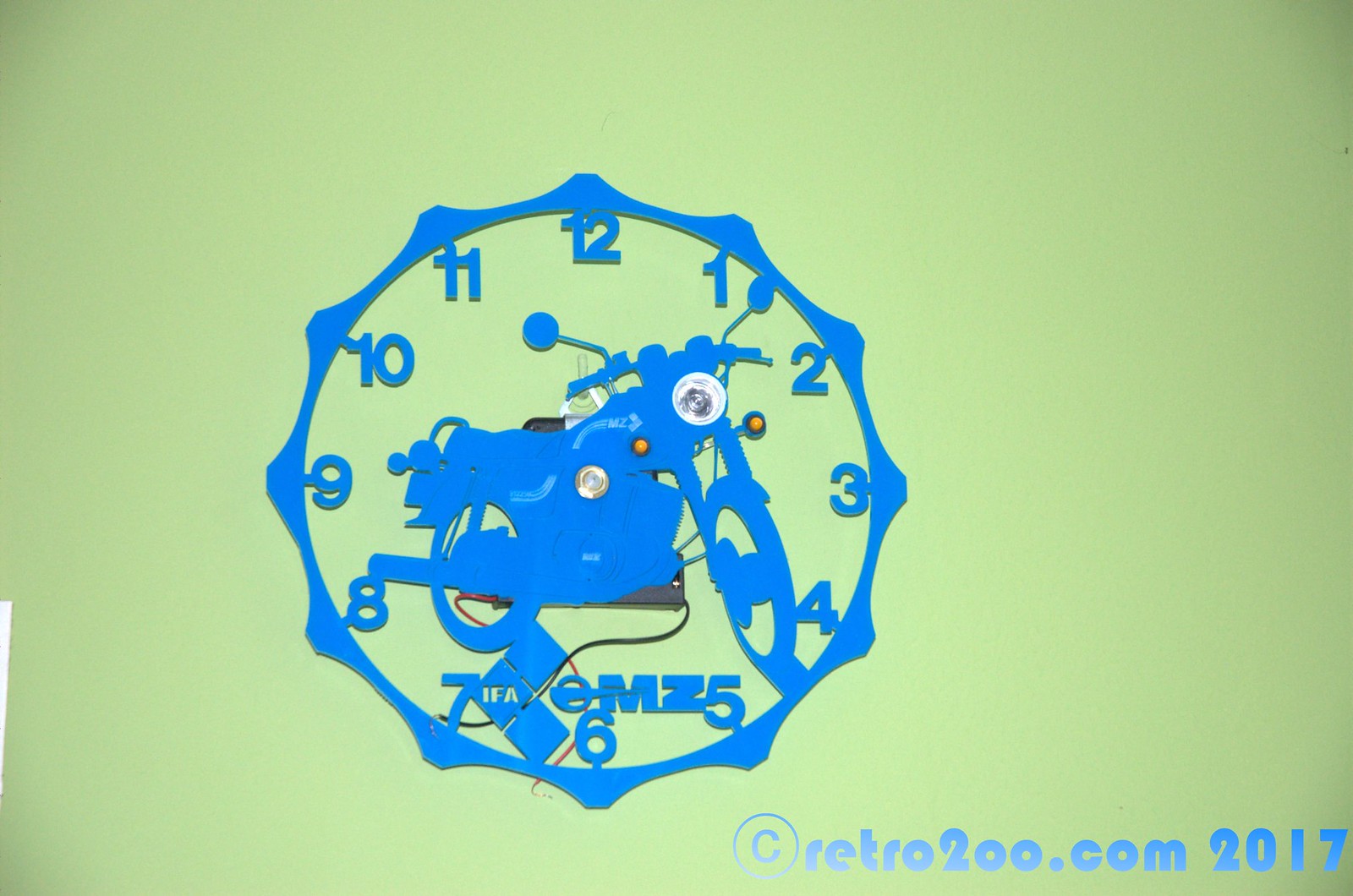A meticulously designed web graphic showcases an intricate clock, characterized by a gear-like frame and boldly centered by a motorcycle. The clock's hands possess an unconventional design, rendering the time difficult to discern. Traditional Roman numerals from I to XII encircle the clock face, maintaining a classic aesthetic. In the bottom right corner, the graphic features the text "retro200.com" alongside the date "2017," subtly anchoring the piece in a specific temporal and digital context.